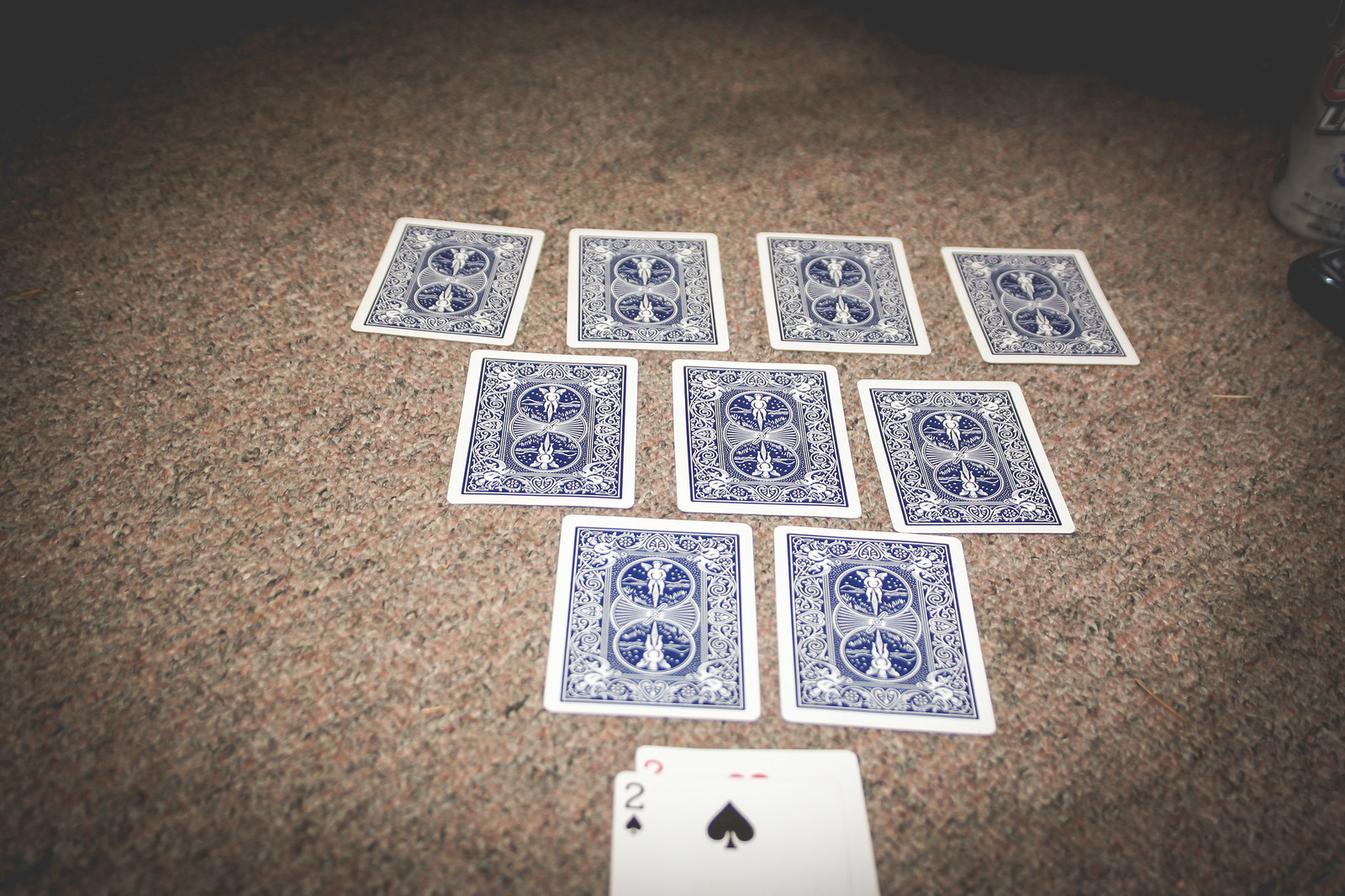The photograph depicts a scattered deck of playing cards arranged on a multicolored, mostly brown and orange Berber carpet. The cards are primarily face down, revealing their navy blue and white backs adorned with an intricate scroll design. Specifically, the cards are laid out in three rows: the first row has four cards, the second row has three cards directly beneath the first, and the bottom row consists of two cards placed beneath the middle row. 

Below the orderly face-down cards, two cards lie face-up. The top card is clearly identifiable as the black Two of Spades, while the card beneath it is partially obscured but appears to be red, possibly another Two, potentially the Two of Hearts – though the exact suit is indiscernible.

The setting is dimly lit, with a circular beam of light, perhaps from a lamp, spotlighting the cards. In the top right corner of the image, an indistinct object is barely visible, its details obscured by the darkness of the room.